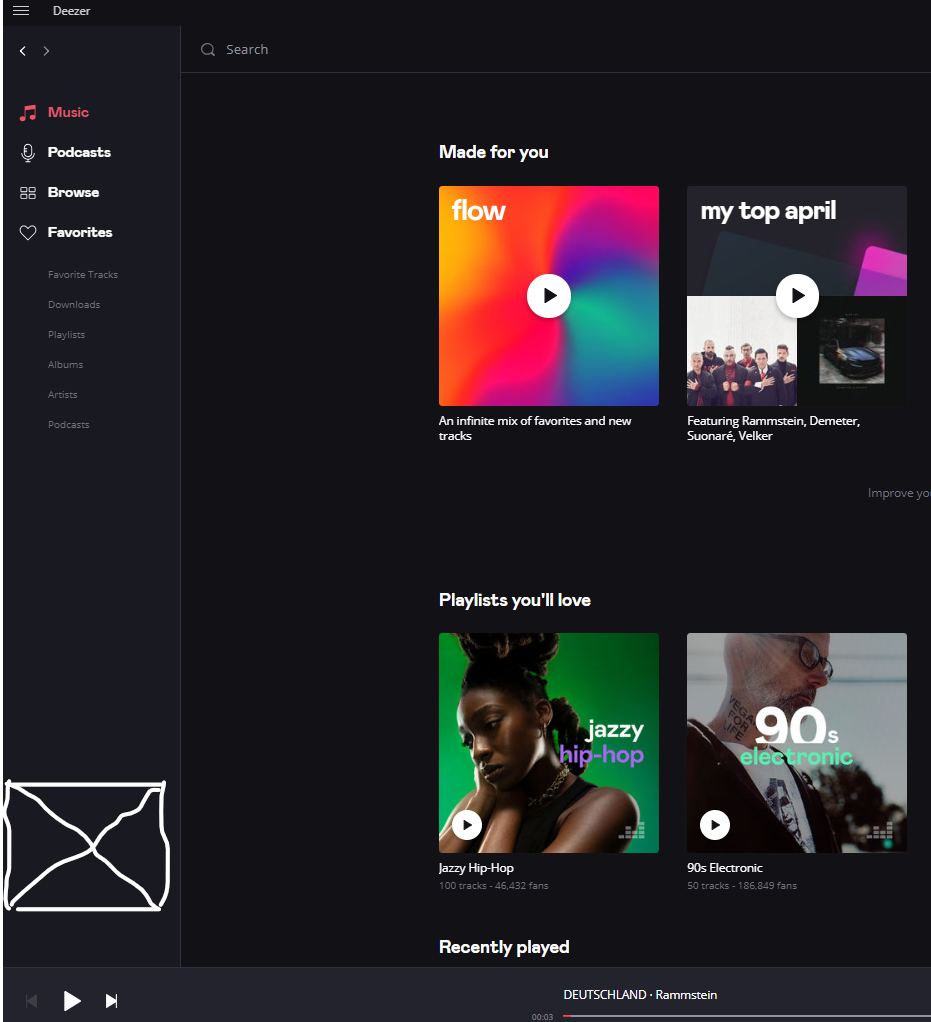A detailed screenshot of a music playing app interface, reminiscent of Spotify. The left-hand sidebar features a vertically listed menu with options such as Music, Podcasts, Browse, and Favorites. Additional options are in smaller, bold white text but are not entirely legible. In the bottom left corner, an added and shaky drawing appears to form a squiggly square with an 'X' through it. Below this doodle are playback controls including back, forward, and play buttons. On the right side, a search bar spans the top, under which four albums are displayed in two rows. The top section, titled "Made For You," includes albums such as "Flow," distinguished by a rainbow design, and "My Top April," showcasing a few highlighted albums. The section below, labeled "Playlists You'll Love," presents album covers including one with a woman on a green background labeled "Jazzy Hip Hop," and another with a man wearing glasses named "90s Electronic."